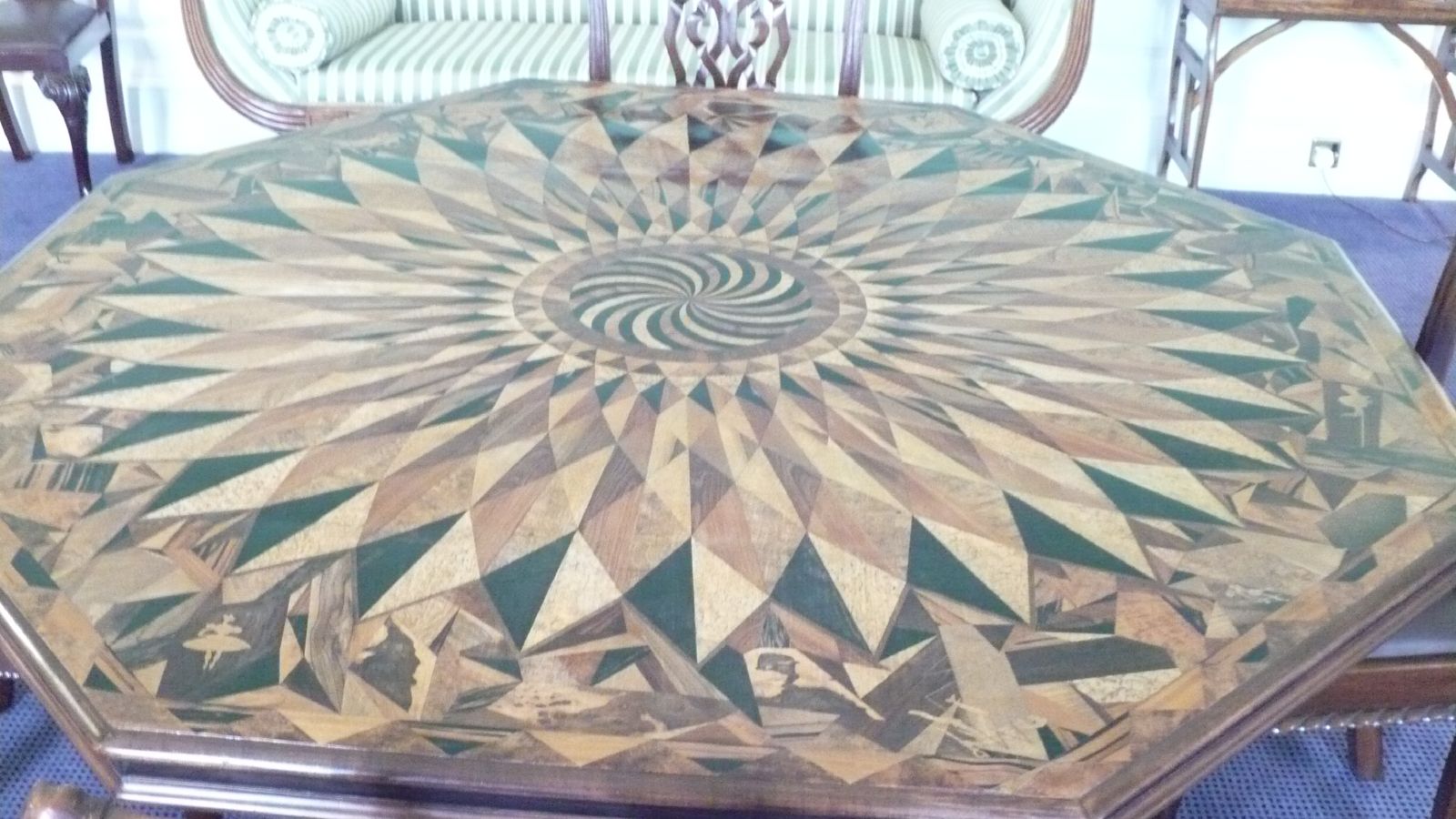The image depicts a wooden octagonal table adorned with an intricate decorative pattern featuring spirals, diamonds, triangles, and lines radiating from a central circle. The tabletop showcases a diverse color palette including black, white, tan, yellowish, almost red, green, light brown, and beige hues. On the sides of the table, there's imagery of ballerinas at the bottom-left corner and the middle of the right side. Surrounding the table, several brown chairs are neatly tucked in, and additional furniture pieces, including two smaller tables, are positioned by the wall. A couch with a green and white striped pattern, wooden frame, and round pillows is situated in the background, accompanied by end tables on either side. The room is finished with a blue or purple carpet underfoot, suggesting the setting is either a well-furnished living room, dining room, or a furniture showroom.